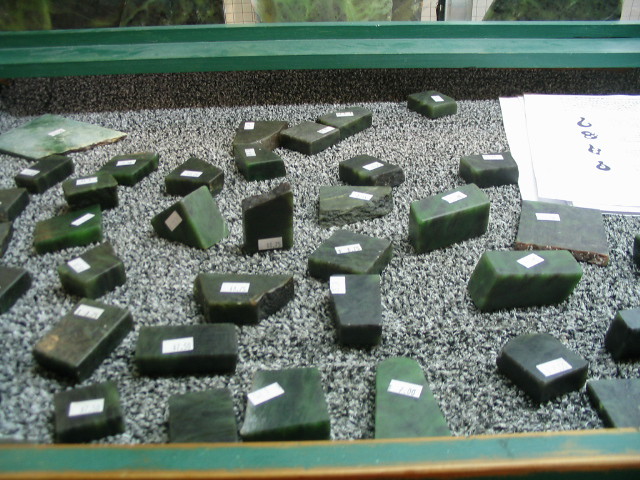The image depicts a display case, possibly in a store, containing an assortment of small green gemstones, with variations in their shapes (some are square, rectangular, and triangular). These green stones, perhaps resembling rough cuts of gemstones, are meticulously arranged within the case, some standing upright while others lie flat or face down. Each gemstone has a white price tag attached, though the prices are not entirely legible from the image, appearing to indicate amounts around $2 to $7. The display case itself is green-bordered and lined with a lighter green carpet-like fabric, blending harmoniously with the stones. Additionally, there's a white piece of paper with foreign lettering visible in the top right corner of the case. The entire scene exudes a predominantly green aesthetic, capturing the attention with its varied shapes and shades of green.